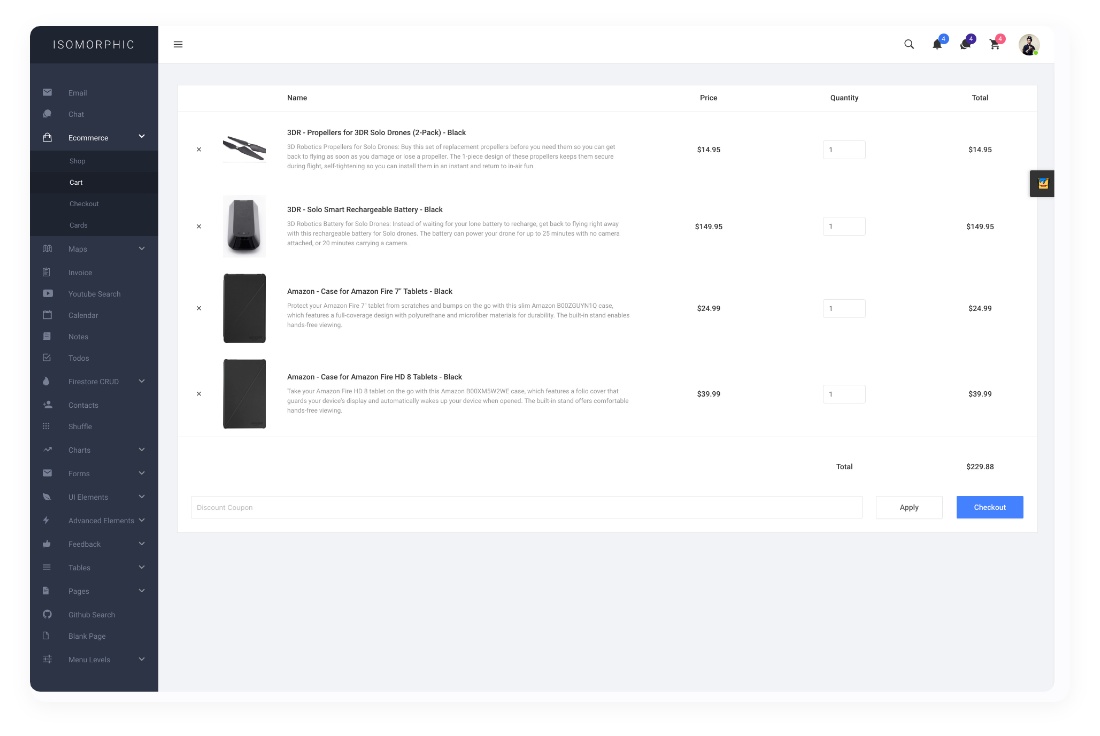The image displays a user interface featuring an "Isomorphic" label on the left side against a dark blue background, which also contains various clickable options that are too small to discern. In the center of the interface, there is a white section labeled with column headers: "Name," "Price," "Quality," and "Year." Below these headers, a long list of items is displayed, including:

- "3BR propellers for 3BR"
- "Silo"
- "Drain"
- "2-pack"
- "Black"
- "Dance Dance Revolution Solo"
- "Smart Rechargeable Battery"
- "Moth"
- "Black"

Further, additional listings related to Amazon Fire tablets are mentioned:
- "Amazon, Corn, for Amazon Fire, 7-inch Tablet, Black"
- "Amazon, Corn, for Amazon Fire HD and Tablet, Black"

The total cost of the items listed amounts to $779.88.